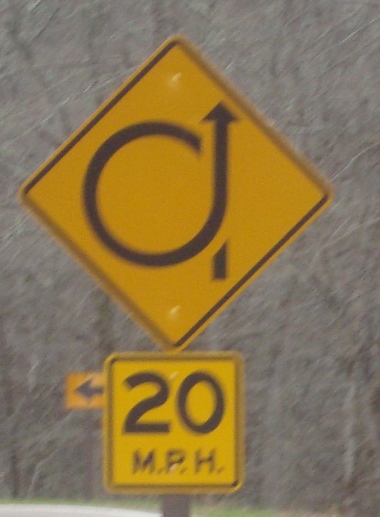This daytime photograph, seemingly captured from inside a vehicle, showcases a roadside signpost against a backdrop of barren trees. The signpost features two signs: a square, yellow sign at the bottom indicating a speed limit of 20 miles per hour, and above it, a diamond-shaped yellow sign displaying a curving arrow that loops into a full circle before straightening out. Additionally, there is an arrow pointing left behind the signpost, visible amidst the dense woodland background composed entirely of leafless trees.